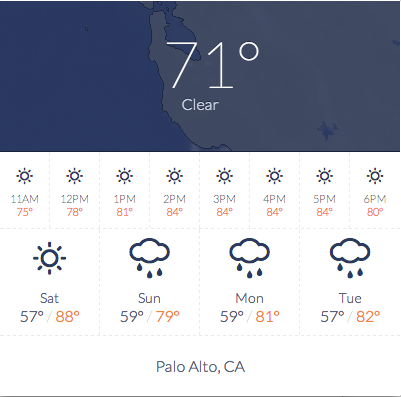This screenshot from a weather app displays the current weather for Palo Alto, California. At the top of the screen, there is a large rectangular box with a dark background and the outline of land faintly visible. Overlaid on this background is the current temperature, "71°," in prominent white lettering, and directly below, the word "Clear" indicating the weather condition.

Below this main heading, there is a timeline forecast spanning from 11 AM to 6 PM, providing hourly weather updates. Further down the page, in dark gray text, it confirms the location as "Palo Alto, California."

At the bottom of the screen, the app provides an extended four-day forecast displayed with larger text and icons, covering the days Saturday, Sunday, Monday, and Tuesday. The detailed presentation of the weather information ensures that users can easily grasp both current conditions and future forecasts at a glance.